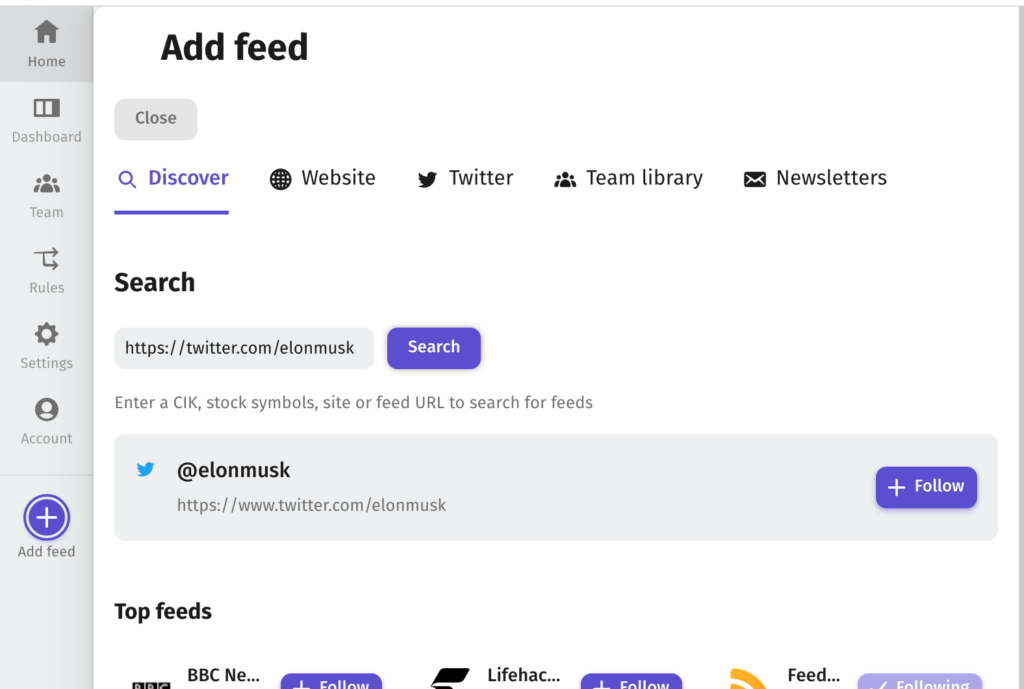The image depicts a web interface with several navigation options and functionalities. Key elements include tabs labeled "Feed," "Home," "Dashboard," and "Team," providing users access to various sections of the site. Additional options like "Rules," "Settings," and "Account" allow for customization and account management. 

Prominent on the interface is the "Add Feed" button, enabling users to integrate new content feeds. Other features include navigational links such as "Close," "Discover," and "Library," as well as access points for "Newsletters" and "Search." 

The interface also includes a section to enter stock symbols, site URLs, or feed URLs to search for specific content feeds. A notable example within the search functionality is a reference to Elon Musk, with a link to his Twitter profile (https://twitter.com/elonmusk) prominently featured. Users are also encouraged to follow top feeds for the latest updates and information.